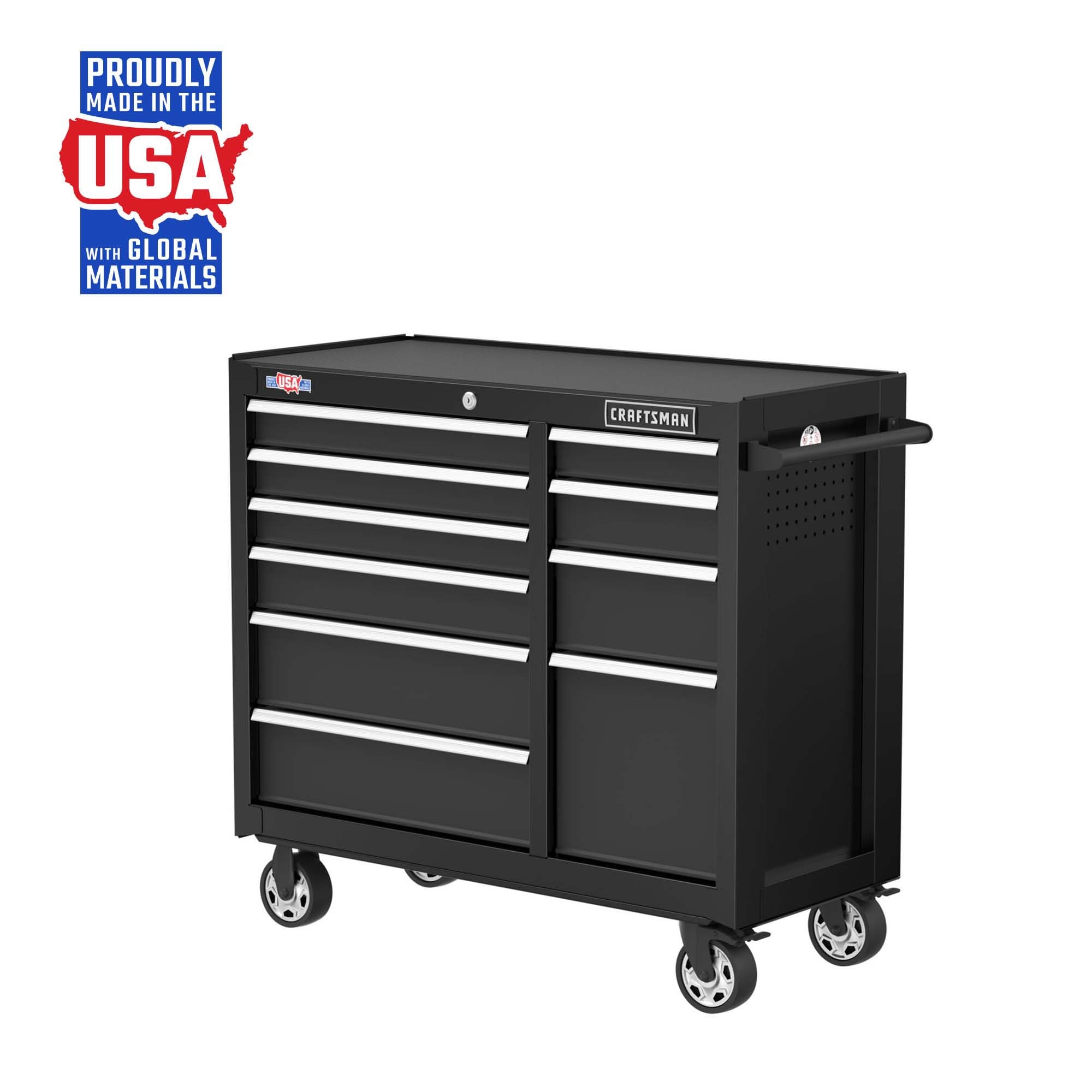This image displays a large, mobile toolbox cart made of metal, designed with a sleek black finish and fitted with four wheels for easy mobility. It features a total of ten drawers of varying sizes, each equipped with white handles that contrast distinctly against the black drawers. On the side of the cart, there is a sturdy handle for pushing. Prominently, the cart brand, "Craftsman," is marked on the front, alongside a bold label stating "Proudly Made in the USA with Global Materials," detailed in red, white, and blue. Additionally, there’s a red outline of the USA adorning the cart, adding to its patriotic design. The cart also includes a lock on the top side for securing the drawers. This detailed setup suggests the image might serve as an advertisement.